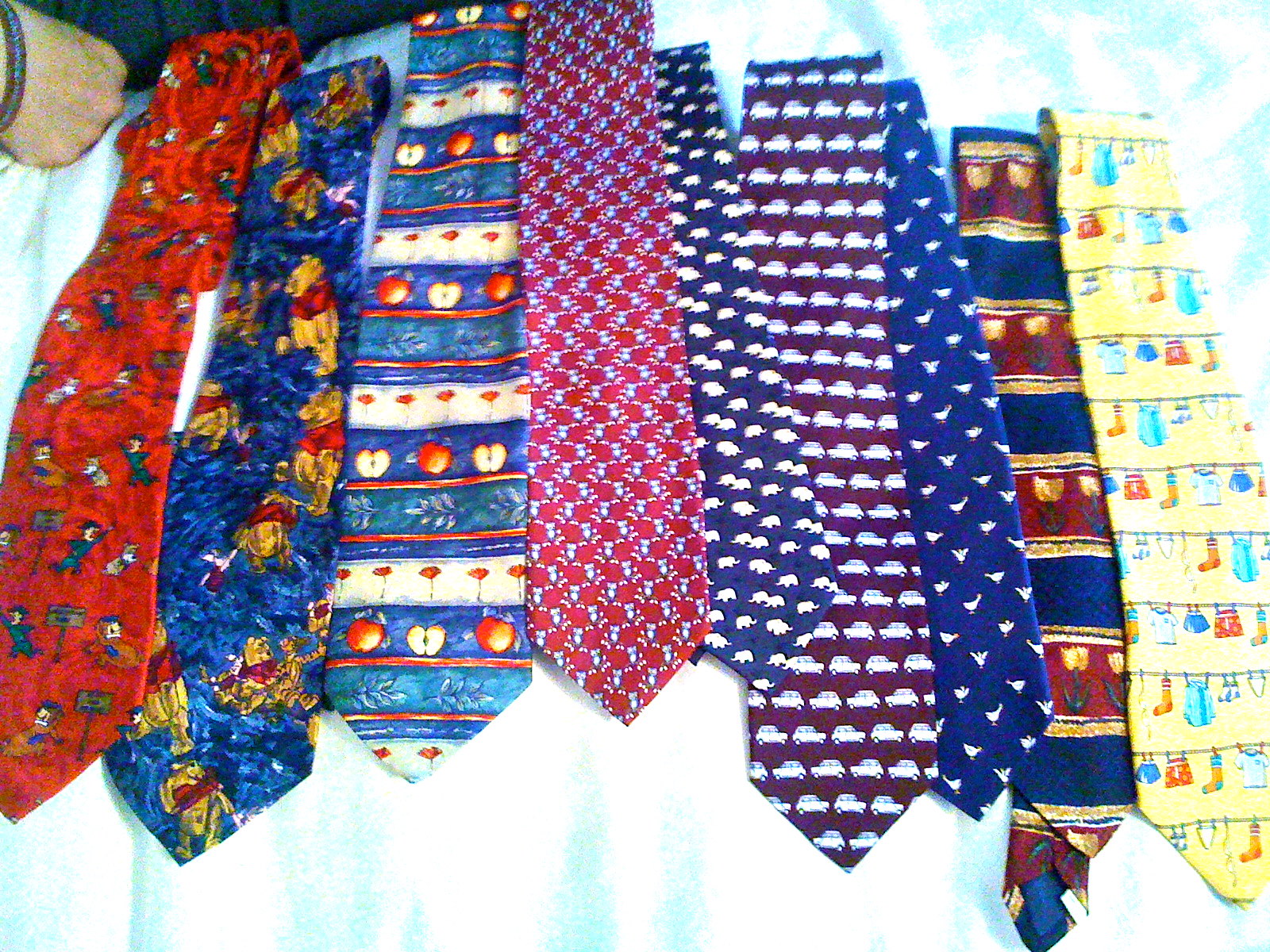The image depicts a collection of nine colorful neckties arranged horizontally on a white and light-blue background, likely a bed sheet. A part of a person’s arm, clad in a blue and white check shirt, is visible in the top left corner, resting on the surface.

From left to right, the ties are:
1. A red tie adorned with small, indistinct cartoon characters.
2. A blue tie featuring several images of Winnie the Pooh.
3. A tie with blue and white stripes, interspersed with red shelves and apple designs.
4. A maroon tie with a light blue, swirly diagonal pattern.
5. A dark blue tie showcasing a subtle pattern of white elephants.
6. A purple tie decorated with small, white car designs.
7. A blue tie displaying small white patterns, possibly birds or abstract shapes.
8. A tie with alternating blue, red, and gold bands featuring floral elements.
9. A bright yellow tie illustrating a clothesline with various hanging garments, such as T-shirts, socks, and shorts.

The overall impression is a collection of whimsical, playful ties, possibly belonging to someone like a teacher, captured in a brightly lit, somewhat overexposed photograph.